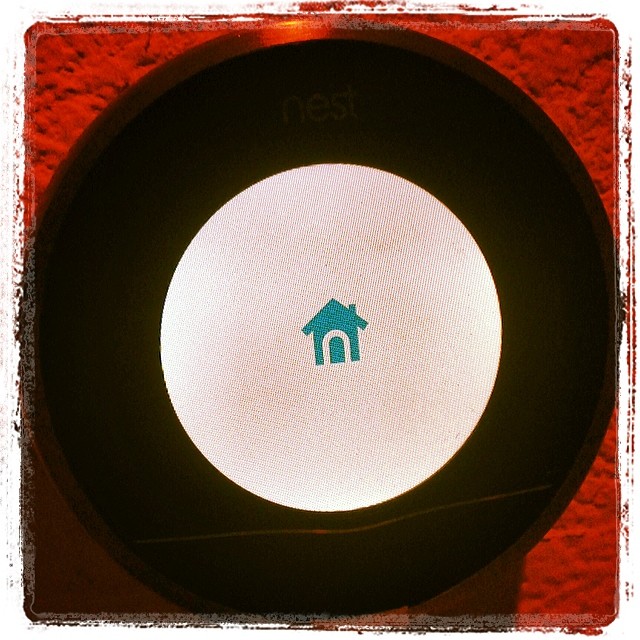This vibrant color photograph showcases a digital thermostat mounted on a red, textured wall. The central focus is a sleek, circular thermostat with a black outer ring that contrasts sharply against the vivid backdrop. Nestled within this black ring is a smaller, white circle that houses a minimalist blue illustration of a house, complete with a roof and an oval front door, suggesting its purpose for home climate control. Intriguingly, the very top of the black ring is subtly illuminated with a faint red light, hinting at an active status or sensor. The photo has a square composition with edges that fade out in a marker-like blur, drawing attention to the thermostat and its rich, tactile surroundings. The image is devoid of any text or human presence, allowing the viewer to focus solely on the device and its intriguing aesthetic.